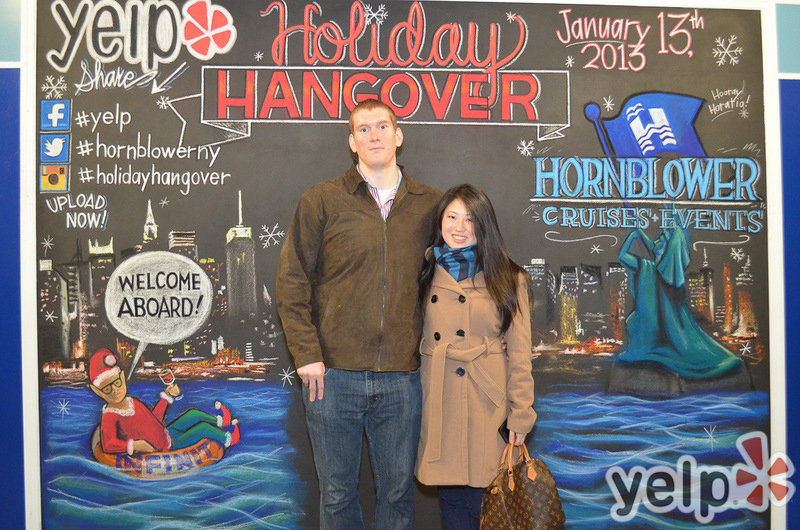In this image, a couple is standing and looking directly at the camera with smiles on their faces. The man, a Caucasian with short auburn hair, is wearing a brown jacket and blue denim jeans. The woman, who appears to be Asian, has hair that falls beneath her shoulders and is dressed in a brownish button-up coat paired with a blue striped scarf. She is also holding a brown handbag. Both are centered in the image, set against a backdrop that features signage with a chalkboard design.

The signage includes multiple elements: in the upper left corner, it says "Yelp" and "Holiday Hangover," dated January 13, 2013. The backdrop also features event details, such as "Hornblower Cruises & Events," and promotional tags "Hashtag Yelp," "Hashtag Hornblower New York," and "Hashtag Holiday Hangover." The words "Upload Now" and "Welcome Aboard" appear in a bubble. The scene appears to depict a holiday-themed event sponsored by Yelp, likely set in a waterway area with a city skyline.

The image also contains various social media logos, suggesting that attendees could share their experiences online. The color scheme includes black, white, red, green, brown, blue, tan, and gray, contributing to the festive and inviting atmosphere of the event.